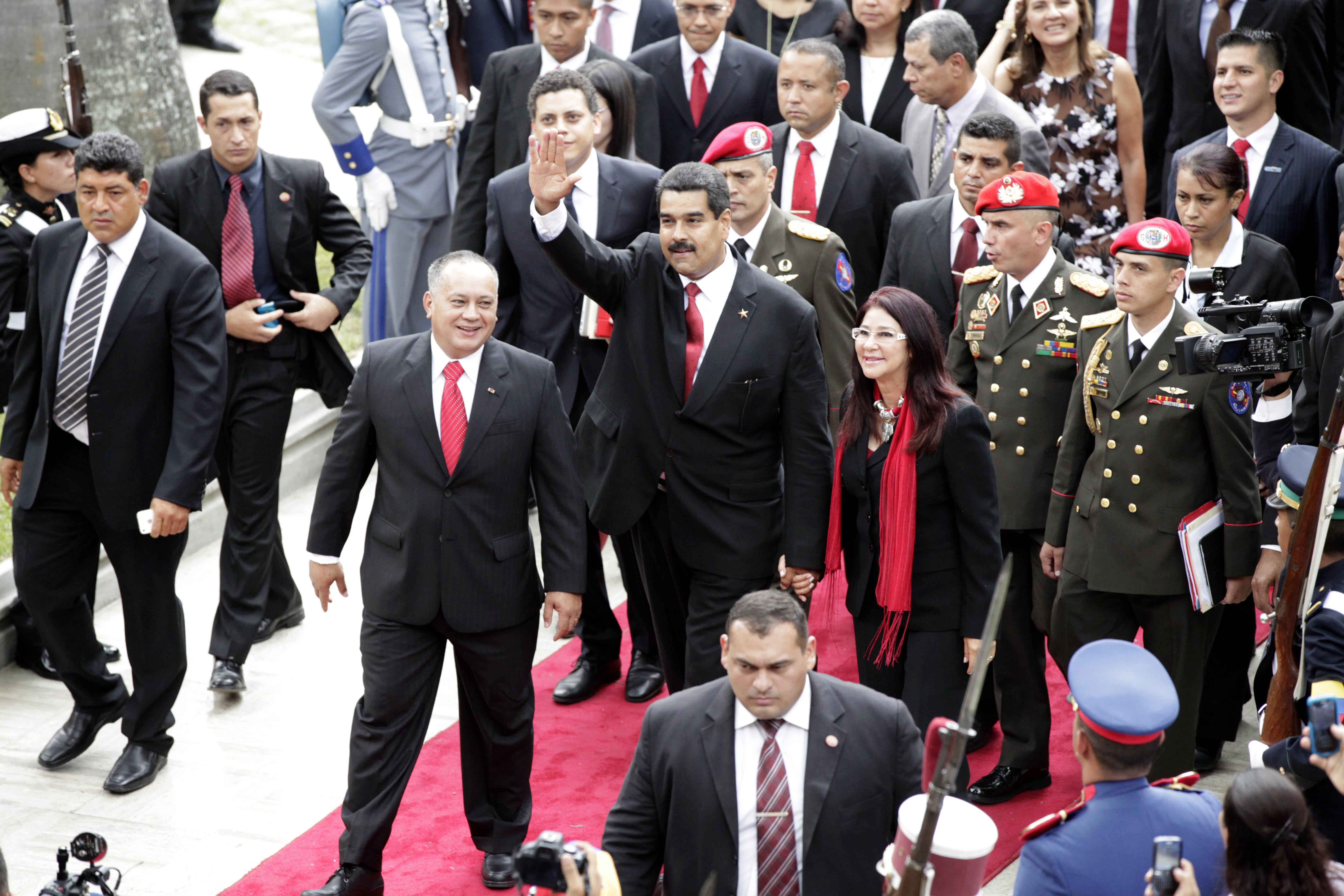The photo depicts a formal event featuring a group of high-ranking officials, most of whom are dressed in black suits with red ties, walking down a red carpet. Central to the image is a man in a black suit and red tie, waving at the camera. Immediately behind him are three high-level military officers wearing red berets, signifying their elite status. Flanking the main group, several lower-level military personnel stand watchfully at the sides, some holding rifles. Beside the central waving gentleman stands a middle-aged woman with brown hair, adorned in a red scarf. In front of this central figure is another gentleman, approximately 50 years old, also dressed in a suit and red tie. The setting and attire of the individuals suggest a significant government-related occasion.